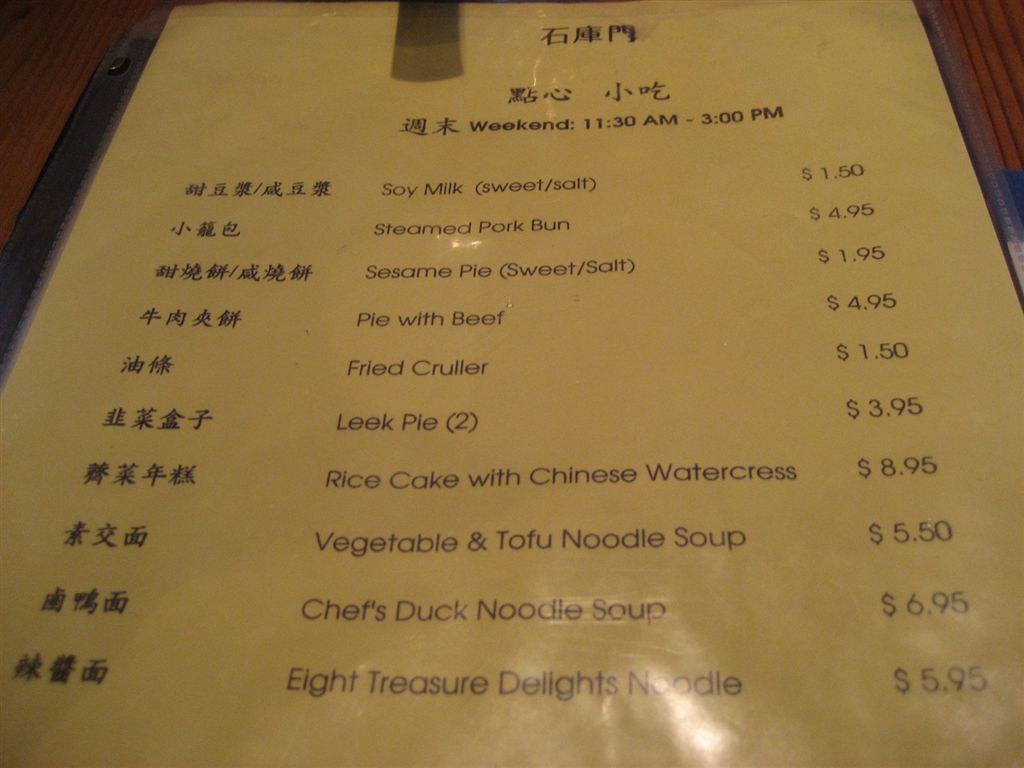In this photograph, a partially visible wooden table occupies the top right corner, showcasing its elegant texture with darker grains running through it, also visible on the left side of the image. The photo prominently features a restaurant's menu printed in black ink, written in a foreign language—possibly Chinese or Japanese—running vertically down the left side. 

Centrally, English descriptions with corresponding prices are listed clearly. The items include:

- Soy Milk (sweet, salt) - $1.50
- Steamed Pork Bun - $4.95
- Sesame Pie (sweet, salt) - $1.95
- Pie with Beef - $4.95
- Fried Cruller - $1.50
- Leek Pie (2) - $3.95
- Rice Cake with Chinese Watercress - $8.95
- Vegetable and Tofu Noodle Soup - $5.50
- Chef Duck Noodle Soup - $6.95

At the top of the menu, foreign characters are arranged in a sequence of three then two, with a space, followed by another two characters. Below these characters, in English, it states "Weekend 11:30 a.m. to 3 p.m."

The clean, minimalist layout in black ink ensures that each item and its price are easily readable, while the detailed foreign script adds an authentic touch to the menu's presentation.